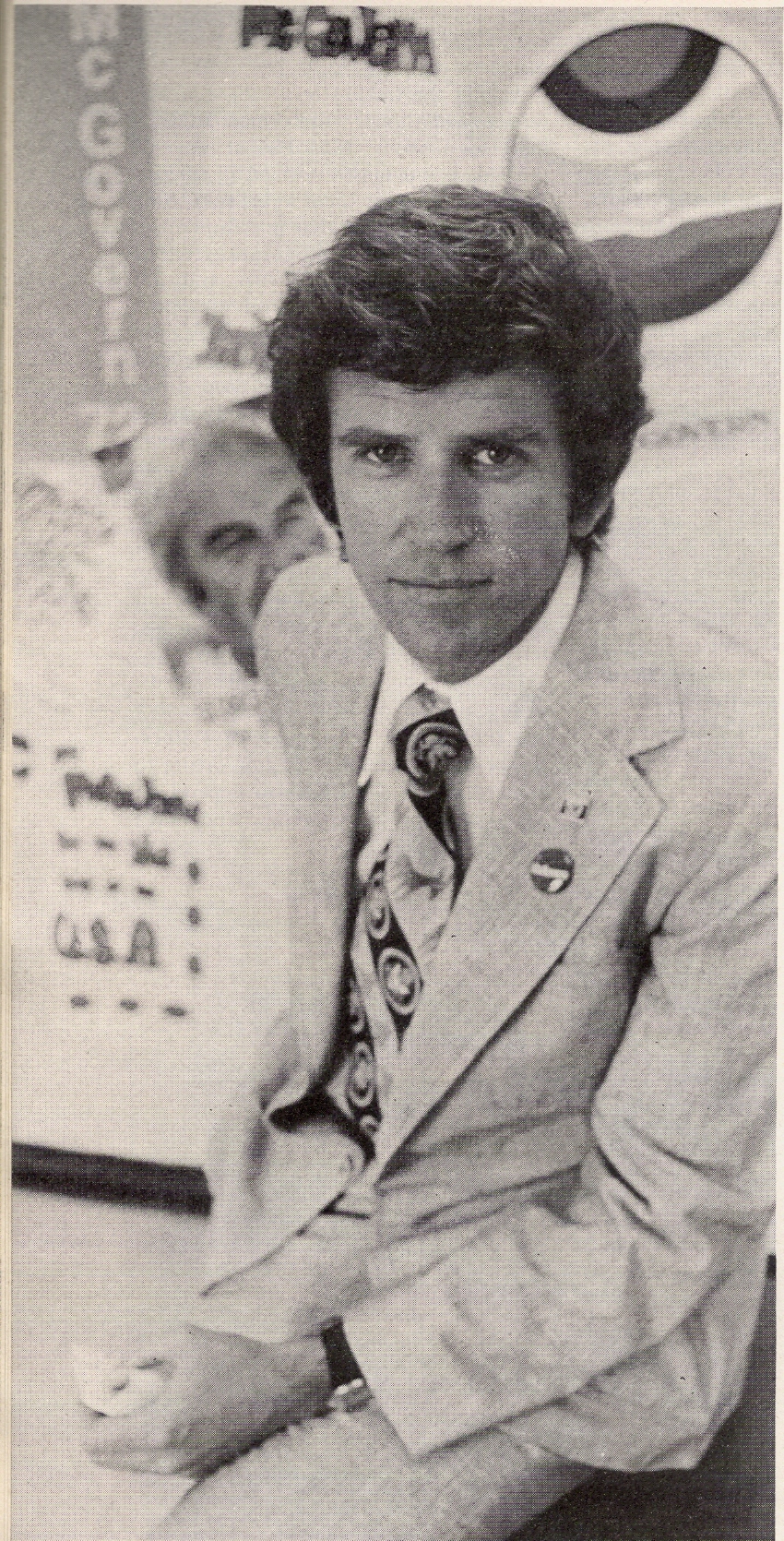In this black and white photograph, a young man with thick, wavy, black hair sits near the right-hand side of the image, looking directly at the camera with a smirk. He wears a suit with a sports jacket and matching pants, a white shirt, and a tie featuring a striped pattern with indistinct logos or animal patterns. His left wrist sports a wristwatch. On his left lapel, there are two pins—a button and a flag pin. He holds a white object, possibly paper, in one hand, resting on his leg. Behind him, partially obscuring his figure, is the face of an older man emerging near his shoulder. The background features a "McGovern 72" sign in the upper left corner, hinting at a political campaign, and a circular emblem on the upper right, possibly depicting a horizon and water scene.